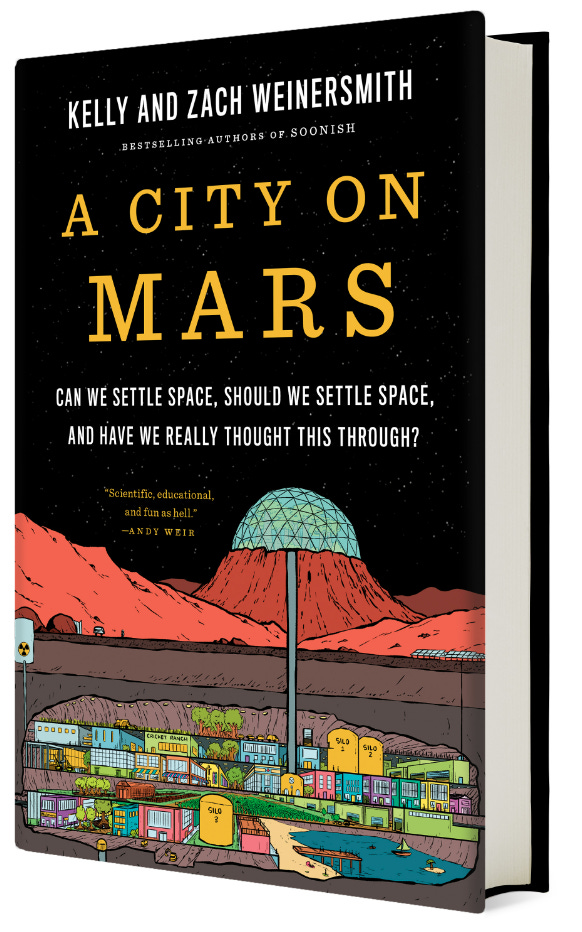The book cover, set against a black background, prominently features the title "City on Mars" in a striking yellow font. At the top, it reads "Kelly and Zach Weinersmith, bestselling authors of Soonish." Beneath the title, the intriguing subtitle asks: "Can we settle space? Should we settle space? And have we really thought this through?" The cover showcases a detailed illustration of a reddish landscape dominated by an orange mountain. Atop this mountain, a green, half-sphere dome with a lead pattern stands out, resembling a crater with a dome built on it. Beneath this is a colorful depiction of various buildings, suggesting a vibrant underground settlement. A blue river, with two boats, flows in the lower right corner, adding depth and life to the scene.